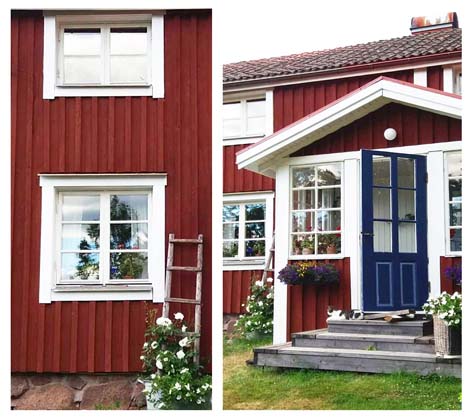The image is a composite of two photos side-by-side separated by a thin white border, showcasing the same red corrugated barn-style house from different angles. The left photo zooms in on the first and second-floor windows, both framed in white with the top window featuring four glass panes and the bottom six. This section has a red metal corrugated siding with vertical lines, supported by a rock and cement foundation. A small wooden ladder leans against the house near a blooming white flower. The right photo offers a wider view, displaying the front of the house which includes a blue door with six glass panes, accessible by three wooden steps. Flanking this entrance are white-trimmed windows and various flowering plants, suggesting this area might be an addition to the main structure. Both images reveal the house's terra cotta roof tiles and a serene garden with vibrant green foliage. A cat sits perched on the top step near the blue door, adding a charming touch to the scene.